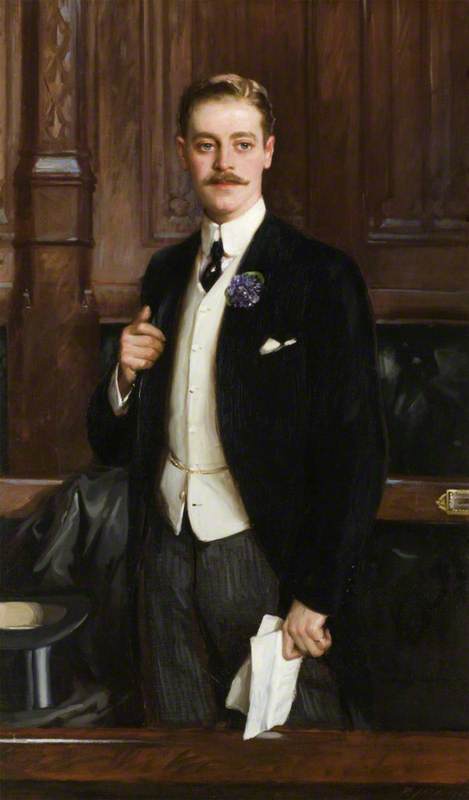A meticulously detailed oil-on-canvas painting showcases a sharply dressed young man, possibly a lawyer or dignitary, standing in the center of a richly paneled room. The walls behind him are adorned with elaborate woodwork and small gold plaques, adding a touch of opulence reminiscent of Baroque or Realist styles. The man gazes directly at the viewer, exuding confidence and sophistication. He dons a long black jacket over a crisp white vest and shirt, accentuated by a white collar and a gold watch chain draped across his waist. In his left hand, he holds two pieces of paper, indicating his professional demeanor. His right hand rests on the handle of a black leather bag, which is placed on a chair beside him. A black top hat is positioned nearby. The room's aesthetic is dominated by shades of brown, from the polished wooden desk in front of him to the overall warm, earthy tones of the interior, creating a harmonious and distinguished atmosphere.